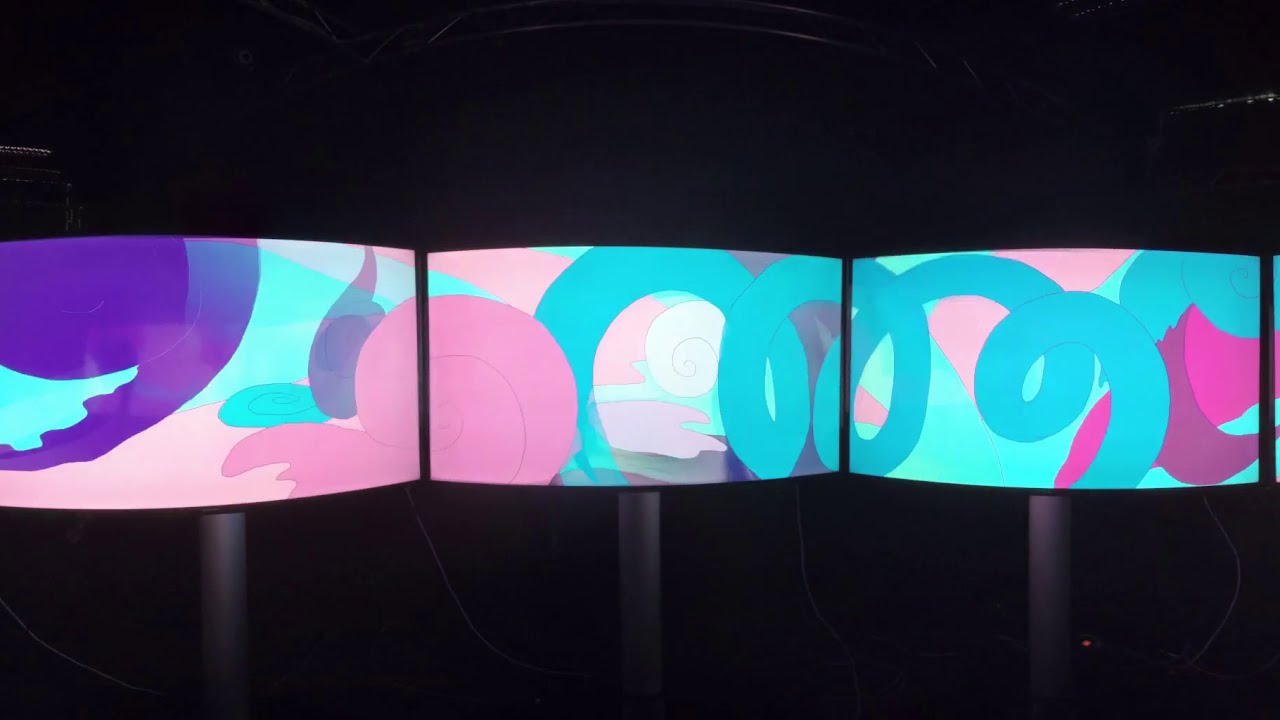The image features three digital screens mounted on gray metal poles, evenly spaced and set against a pitch-black background. These horizontal, rectangular screens are arranged in a row, each displaying a unique yet interconnected swirling design that flows seamlessly from one screen to the next. Starting from the leftmost screen, vibrant swirls of purple and blue blend into pinks, forming a cohesive image that extends across the middle screen where pinks dominate, mingling with turquoise hues. This color scheme continues onto the rightmost screen, with light pinks, dark pinks, and shades of blue swirling and looping to complete the entire vibrant display. The intricate patterns on the screens include swirls, slashes, and feather-like elements, creating a mesmerizing and fluid design that integrates each screen into a single, harmonious artwork.